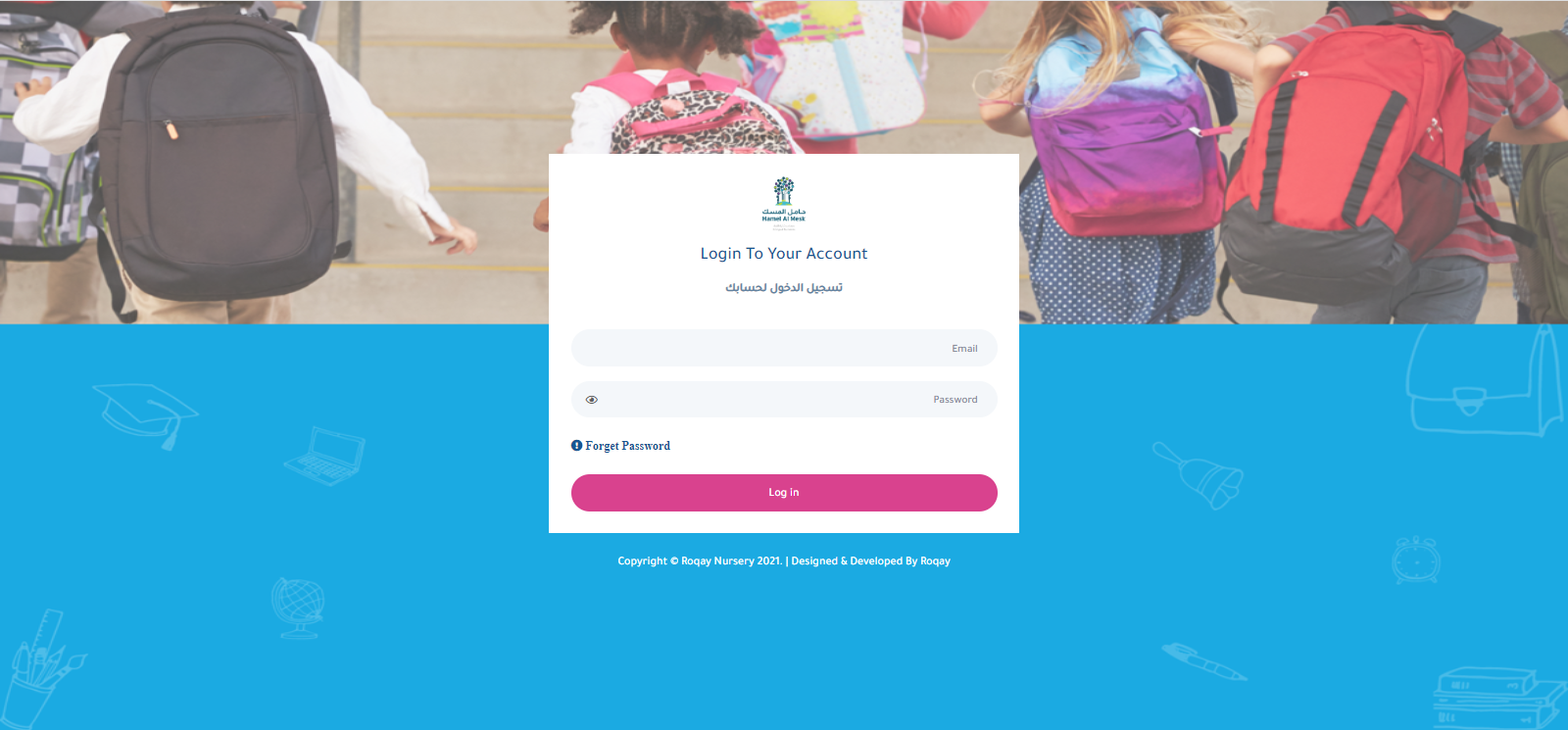The image showcases a cheerful morning scene of young elementary school children, each wearing colorful backpacks, enthusiastically running up a set of steps towards their school. Their joyful expressions suggest their excitement and eagerness to start the school day.

In the foreground, there's a blue rectangle bar at the bottom filled with cartoon-style icons depicting elements of school life, such as a graduation cap, a laptop, a globe, a school bell, a book bag, a clock, a stack of books, and a pen. Above this, a white text box stands out prominently, inviting users to "log in to your account."

This white login section includes fields for entering an email and password, with a "forgot password" link accompanied by a blue exclamation-mark icon. The pink, rounded login button adds a touch of color, making the login prompt user-friendly and noticeable. At the bottom of the image, it indicates the website's copyright information, "© Roque Nursery 2001," and notes the site's design and development by "Roquay," stylized as "R-O-Q-A-Y."